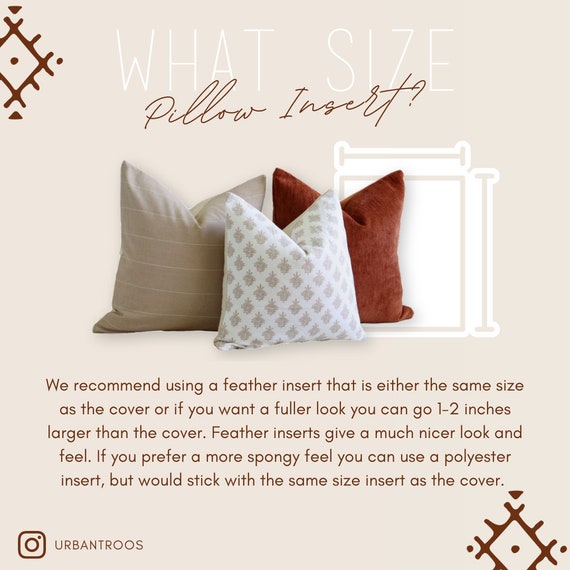The image is an advertisement with a tan background featuring three upright pillows of different designs: a light brown with white stripes, a white pillow with a brown diamond pattern, and a dark red pillow. At the top of the ad, text in white reads "What size," and below it, in cursive brown text, reads "pillow insert." Brown squiggly lines form diamonds with dots at their centers and corners in the top left and bottom right corners of the ad. The middle section features the pillows arranged in a row. Below the pillows, brown text recommends using a feather insert the same size as the cover or one to two inches larger for a fuller look, noting that feather inserts provide a nicer look and feel. For a spongy feel, polyester inserts are suggested, but it's recommended to stick to the same size as the cover. The bottom left corner features a brown Instagram logo followed by the name Urban Truce.